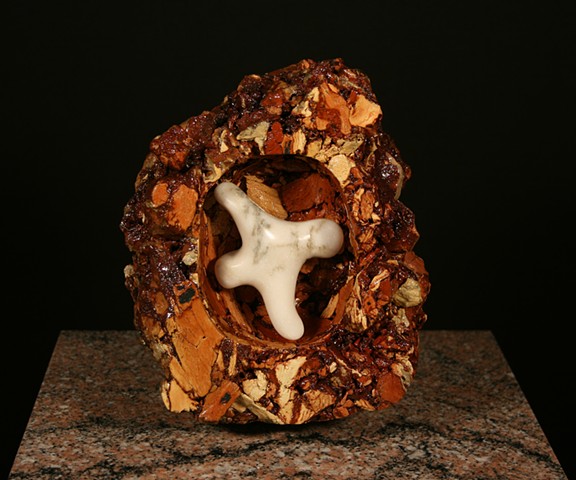The photograph showcases an intricate piece of art set against a black background, accentuating its detailed craftsmanship. The centerpiece is a rock with striking red, yellow, and orange hues, presenting a vivid contrast of dark reds, browns, and oranges. This rock is meticulously hollowed out to reveal an embedded object. Inside, a light beige to white, marble-like figure is carefully placed. This figure, resembling a star or a headless humanoid with two legs and two arms, has a smooth, polished finish. The rock and its internal figure rest on a square slab of what appears to be marble or granite countertop, adding a further layer of visual intrigue with its pristine surface. The entire composition is a compelling blend of color and texture, highlighting the contrast between the rough, vibrant outer rock and the smooth, pale inner form.